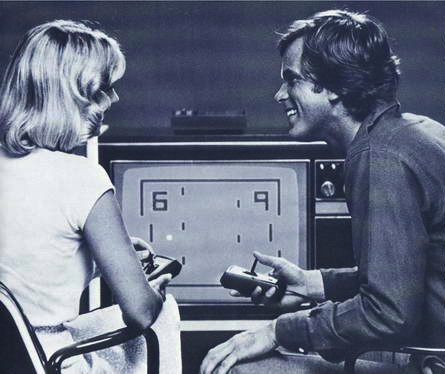This black and white photograph, reminiscent of the late 1970s or early 1980s, depicts a nostalgic scene featuring a couple seemingly engaged in a vintage video game session. Set against a stark dark background, the image captures the duo seated side-by-side in black chairs. On the left, a woman with short, dirty blonde hair is dressed in a short-sleeved white top or dress. She's holding a joystick in her left hand, her back facing the viewer. To her right, a man with dark, possibly brown hair, and clad in a long-sleeved dark shirt, is pictured in side profile, smiling or laughing while gazing at her. He has a similar joystick in his right hand. The background reveals an old-style TV set, its black frame contrasting with the gray screen that displays the game Pong. On the screen, simple black pixelated numbers show that the woman has a score of 6, while the man has a score of 9. This candid moment, rich in detail, evokes a sense of delight and fondness for the early era of home video gaming.